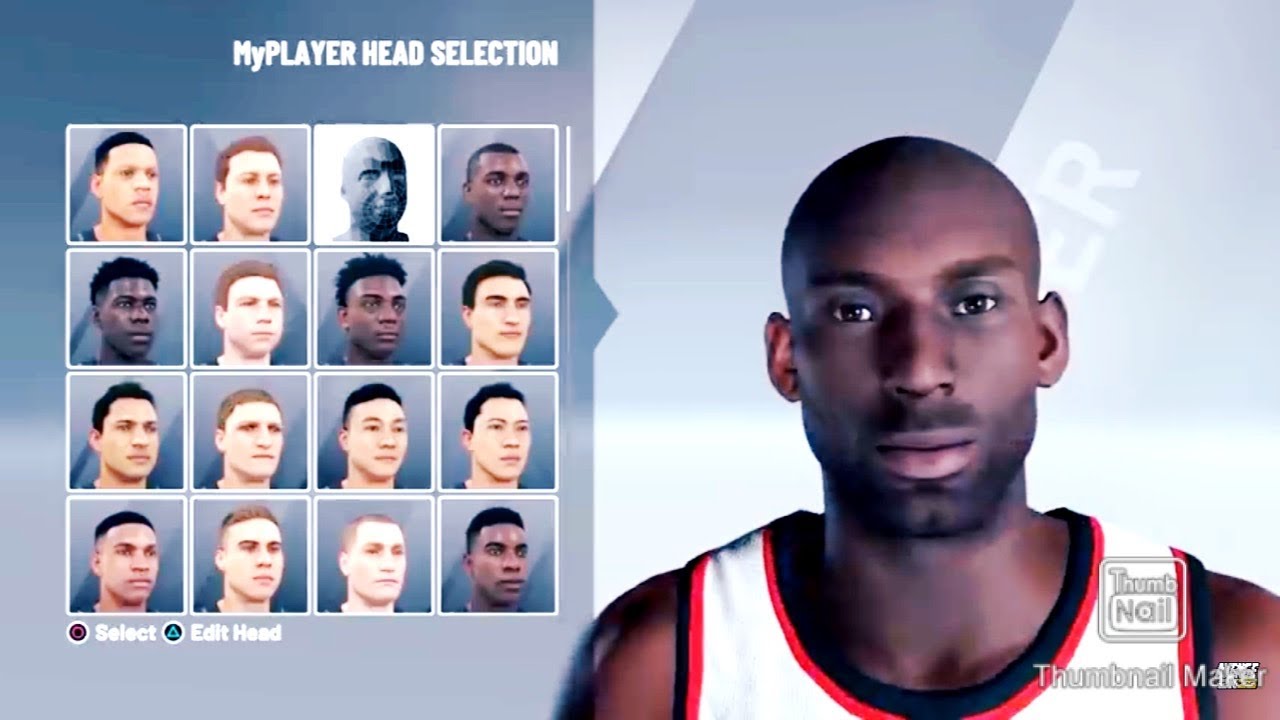This image depicts a catalog of characters, possibly from a video game, displayed in a grid format. There are four squares horizontally and four squares vertically, making a total of 16 character portraits. The art style appears more graphic than realistic. Here’s a detailed breakdown of each character from the catalog:

1. **First Row, First Column**: A light-skinned male character with black hair.
2. **First Row, Second Column**: A light-skinned character with brown hair.
3. **First Row, Third Column**: A character whose appearance resembles that of carved stone; its humanity is ambiguous.
4. **First Row, Fourth Column**: A dark-skinned character with black hair and a haircut.

5. **Second Row, First Column**: The highlighted character, which shows a larger image to the right of the grid, matching the appearance and details of one of the characters in the frames.
6. **Second Row, Second Column**: A character with long, black hair.
7. **Second Row, Third Column**: A light-skinned character with brown hair.
8. **Second Row, Fourth Column**: A dark-skinned character with long hair.

9. **Third Row, First Column**: A light-skinned character with black hair.
10. **Third Row, Second Column**: Another light-skinned character with black hair.
11. **Third Row, Third Column**: A light-skinned character with gray hair, potentially with unusual styling.
12. **Third Row, Fourth Column**: Yet another light-skinned character with black hair.

13. **Fourth Row, First Column**: A light-skinned character with black hair featuring a side cut.
14. **Fourth Row, Second Column**: A light-skinned character with gray hair.
15. **Fourth Row, Third Column**: Another light-skinned character with gray hair.
16. **Fourth Row, Fourth Column**: A dark-skinned character with black hair.

The image showcases a variety of character designs, with differences in skin tone, hair color, and hair style, reflecting a diverse cast that users can presumably select or interact with in the game.